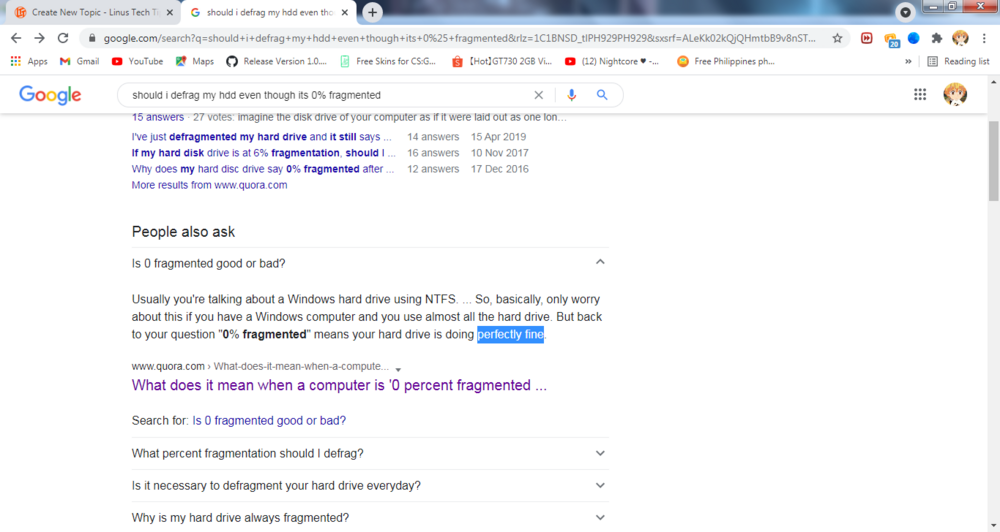The image depicts a web browser window with two tabs open at the top. The first tab is titled "Create New Topic - Tech" and the second tab is partially titled "Should I defrag my HDD even though." The active web page is loaded in the browser, displaying navigation options including a left arrow, a right arrow, and a refresh button. The address bar is populated with a URL, accompanied by a star icon and some graphical elements to its right.

Below the navigation bar, a bookmarks or apps bar is visible, listing various items such as "Apps," "Gmail," "YouTube," "Maps," "Release version 1.0," "Free skins for CSG," "Free Philippines PH," and "YouTube 12 Nightcore."

The main content of the web page consists of a Google search results page for the query: "Should I defrag my HDD even though it's 0% fragmented." The search results include several blue-link entries such as:
- "I defragmented my hard drive and it still says 0% fragmented."
- "If my hard drive is at 6% fragmentation should I..."
- "Why does my hard disk drive say 0% fragmented after..."

Further down, a "People also ask" section features questions like:
- "Is 0% fragmented good or bad?"
- "What does it mean when a computer is 0% fragmented?"
- "What percent should I defrag?"
- "Is it necessary to defrag your hard drive every day?"
- "Why is my hard drive always fragmented?"

These entries are accompanied by brief answers and options for additional searches related to hard drive fragmentation and maintenance.